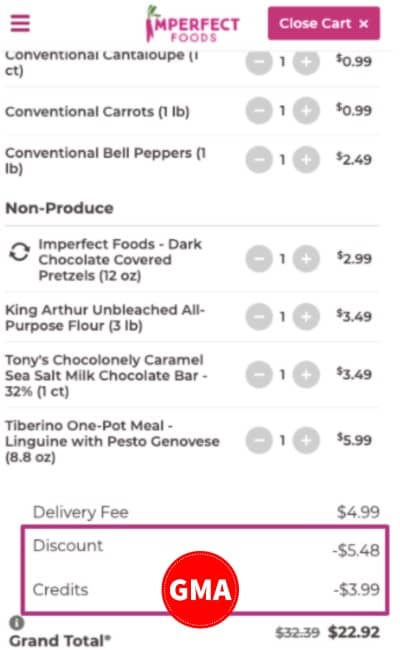The image features a white background with various elements in purple. To the left, there is a purple hamburger icon, and next to it is a purple square containing a white shopping cart and an "X" symbol. The upper text reads "Imperfect Foods" in purple.

Below, the image details various grocery items with their respective names, quantities, and prices:

- Conventional Carrots: 1 lb (0.99 cents) - Each item has a "1" to start, with a plus (+) and minus (-) sign on either side for adjusting the quantity.
- Conventional Bell Peppers: 1 lb ($2.49)
- Non-Produce Item: Displays a refresh symbol
- Imperfect Foods Dark Chocolate Covered Pretzels: 12 oz ($2.99)
- King Arthur Unbleached All-Purpose Flour: 3 lb ($3.49)
- Tony's Chocolate Caramel Sea Salt Milk Chocolate Bar: 32% Cocoa, 1 count ($3.49)
- Turbiny One Pie Meal Linguine with Pesto Genovese: 8.8 oz ($5.99)

At the bottom, it mentions a delivery fee of $4.99 and highlights a purple rectangle around "Discount and Credits."